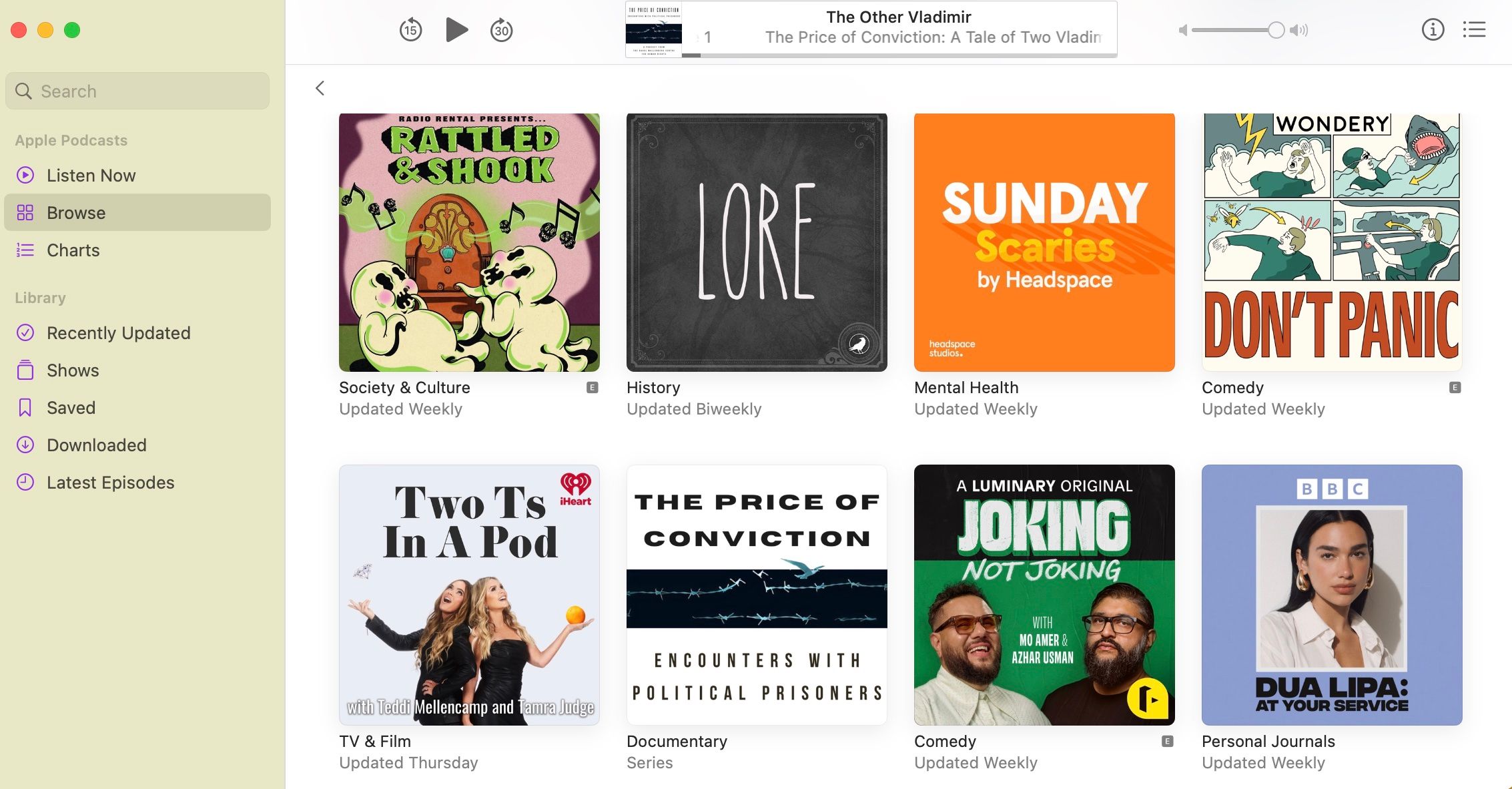Landscape-oriented screenshot of a laptop or computer featuring a podcast collection. The left side displays a beige column with red, yellow, and green circles at the top left. Below these circles, the interface includes a search bar followed by the heading "Apple Podcasts" and options such as "Listen Now," "Browse," and "Charts" marked with pink icons. Further down, a gray header labeled "Library" leads to categories like "Recently Updated," "Shows," "Saved," "Downloaded," and "Latest Episodes," also identified with pink icons.

To the right, the main section showcases different available podcasts. The first listed is "Rattleton Shook" under the Society and Culture category. Next is "Lore," categorized under History. Following is "Sunday Scaries by Headspace" in the Mental Health category, and "Wondery, Don't Panic" listed under Comedy. The subsequent listings include "Two Ts in a Pod" under TV and Film, "The Price of Conviction" categorized as a Documentary, "Luminary, Joking, Not Joking" under Comedy and noted as being updated weekly, and "BBC, Dua Lipa, At Your Service" listed under Personal Journals, also updated weekly.

At the top of the interface, a currently playing podcast is displayed: "The Other Vladimir" from "The Price of Conviction," specifically the episode titled "A Tale of Two Vladimirs," shown within a white bordered area with black text.